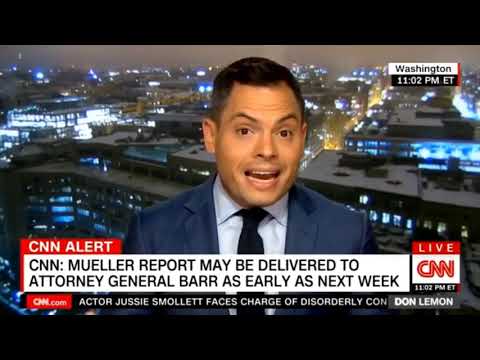The screenshot from a CNN broadcast shows newscaster Don Lemon in the middle of speaking, set against a nighttime backdrop of Washington, D.C. In the upper right corner, the dateline "Washington" and the timestamp "11:02 p.m. Eastern Time" are displayed. A prominent banner at the bottom reads "CNN ALERT: Mueller Report may be delivered to Attorney General Barr as early as next week," with the CNN logo and "Live" indicator beside it. Beneath this, a headline scrolls across the screen stating, "Actor Jesse Smollett faces charge of disorderly conduct." Don Lemon, wearing a blue suit and tie, is captured mid-speech with his mouth open and eyebrows raised. The shared emphasis across the captions highlights the key details: the location, time, important news concerning the Mueller Report, and the additional headline about Jesse Smollett.